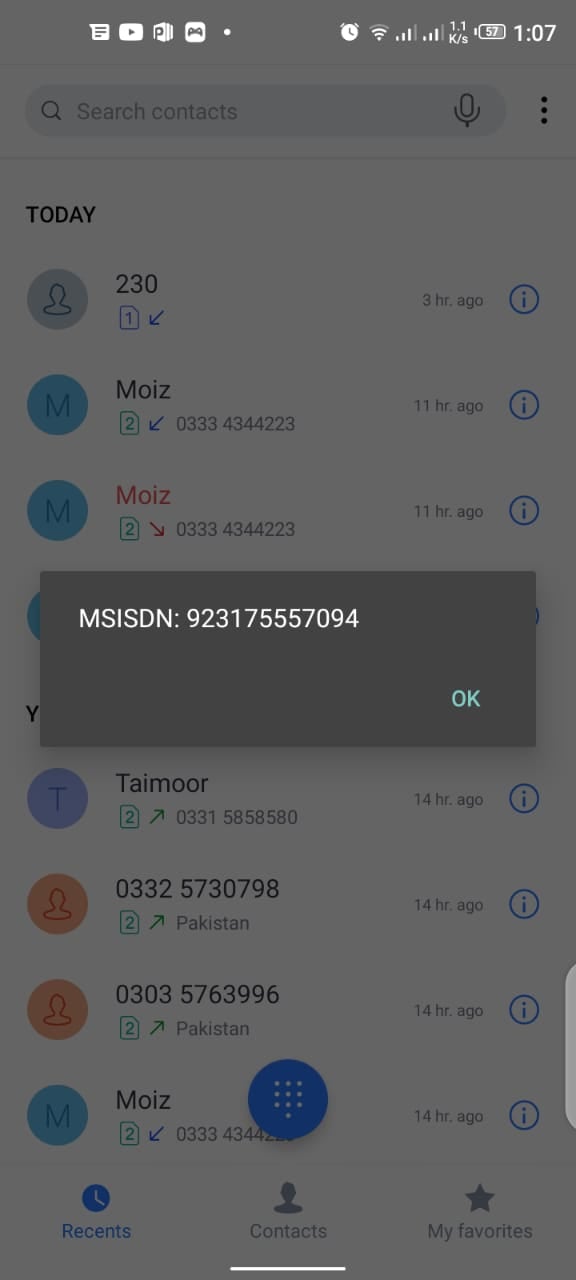A detailed mobile phone screenshot displaying various interface elements. At the top of the screen, white status icons are visible, indicating Wi-Fi connection, alarm status, network signal strength, battery life, the current time, and several app notifications. Near the bottom of the image, there are three navigational buttons: Recents, Contacts, and Favorites. The Recents tab is currently selected, revealing a list of recent contacts within the user’s phone. 

A search bar sits at the top of the Recents list, allowing for quick contact searches. Below the search bar, today's list of recent contacts is shown. The screenshot also features a translucent overlay due to an active pop-up notification.

The pop-up, a dark grey box, contains the text "MSISDN:: 923175557094" and provides an "OK" button to close this notification. The combination of these elements captures a detailed snapshot of a mobile phone's interface at a given moment.